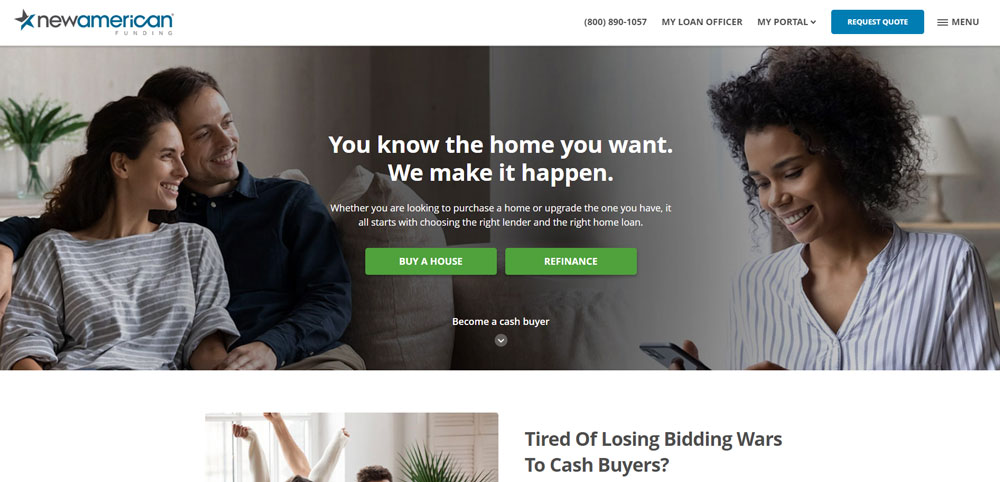The image features a detailed advertisement for "New American Funding." 

At the top left, the text “New American” is styled with "New" in black and "American" in blue, and directly below it, "Funding" is displayed in smaller gray text. Adjacent to this, a black and blue star icon is visible. 

On the right side, there is a phone number followed by the labels "My Loan Officer" and "My Portal" with a downward arrow. A prominent blue button labeled "Request Quote" in white text is situated next to it, and there's an indication for "Many" nearby.

The central image captures a cheerful couple seated on a gray couch. The man is wearing a blue shirt, and the woman is in a gray and white striped shirt. Both are smiling and looking towards the right, with a green plant in a vase behind them adding a touch of nature to the scene.

To the right of this couple, another woman is seen smiling and looking down at her phone. In the center of the image, an inspiring message reads: "Know the home you want, we make it happen. Whether you are looking to purchase a home or upgrade the one you have, it all starts with choosing the right lender and the right home loan."

Below this message are two green buttons: one on the left saying "Buy a House" and the other on the right saying "Refinance." In white text below these buttons, it states "Become a Cash Buyer." Following this, a question poised in white asks, "Tired of losing bidding wars to cash buyers?" The visual concludes with a partially cut-off image of people raising their hands, suggesting a competitive bidding scenario.

This comprehensive depiction of the advertisement effectively combines informative content with inviting visuals to attract potential home buyers or individuals looking to refinance.